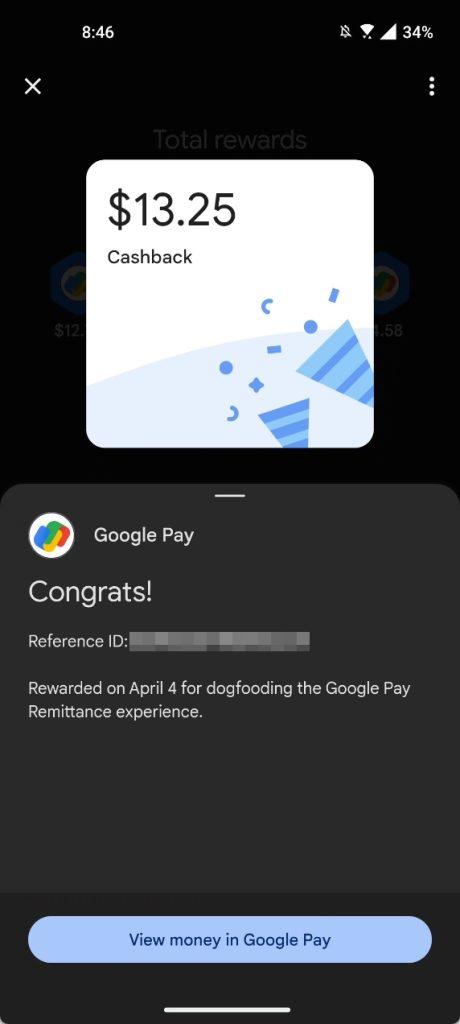The image is a screenshot taken on a smartphone using dark mode, resulting in a predominantly black backdrop with a gradient transition to gray at the bottom. 

At the very top-left corner, "8:46" is displayed in white text, indicating the time. Over to the top-right are several icons in white: a bell with a line through it (a notification mute icon), followed by the Wi-Fi signal strength icon, then the phone signal strength icon, and finally a battery icon showing "34%".

Below this status bar, on the main content area, the screen is segmented into two parts, divided by a white box at the center. 

The top section of the screen features, on the left, a white 'X' icon. On the right are three vertically aligned dots representing a menu.

The central white box is highly detailed. In the top-left corner inside this box, there is a dollar symbol followed by "13.25" in black text. Next to this, the words "Cashback" are also in black. In the bottom right of this box, two colorful confetti poppers are depicted, resembling party hats with blue confetti streaming out.

Below the white box, the background shifts to gray. In the upper left-hand corner of this gray section, there is a circular icon adorned in blue, green, yellow, and red ribbon-like designs. To its right, the text "Google Pay" is written in white. Beneath this, the text "Congrats!" is enthusiastically displayed in white. Following this, there's a section that begins with "Reference ID," but the actual ID is blurred out in white and gray for privacy.

Further down, it reads "Reward on April 4 for dogfooding the Google Pay," and directly below this, "remittance experience" is mentioned in white text.

At the very bottom of the screen, a blue bar stretches across the width. Inside this bar, in a slightly darker shade of blue, the text "View money in Google Pay" is prominently displayed.